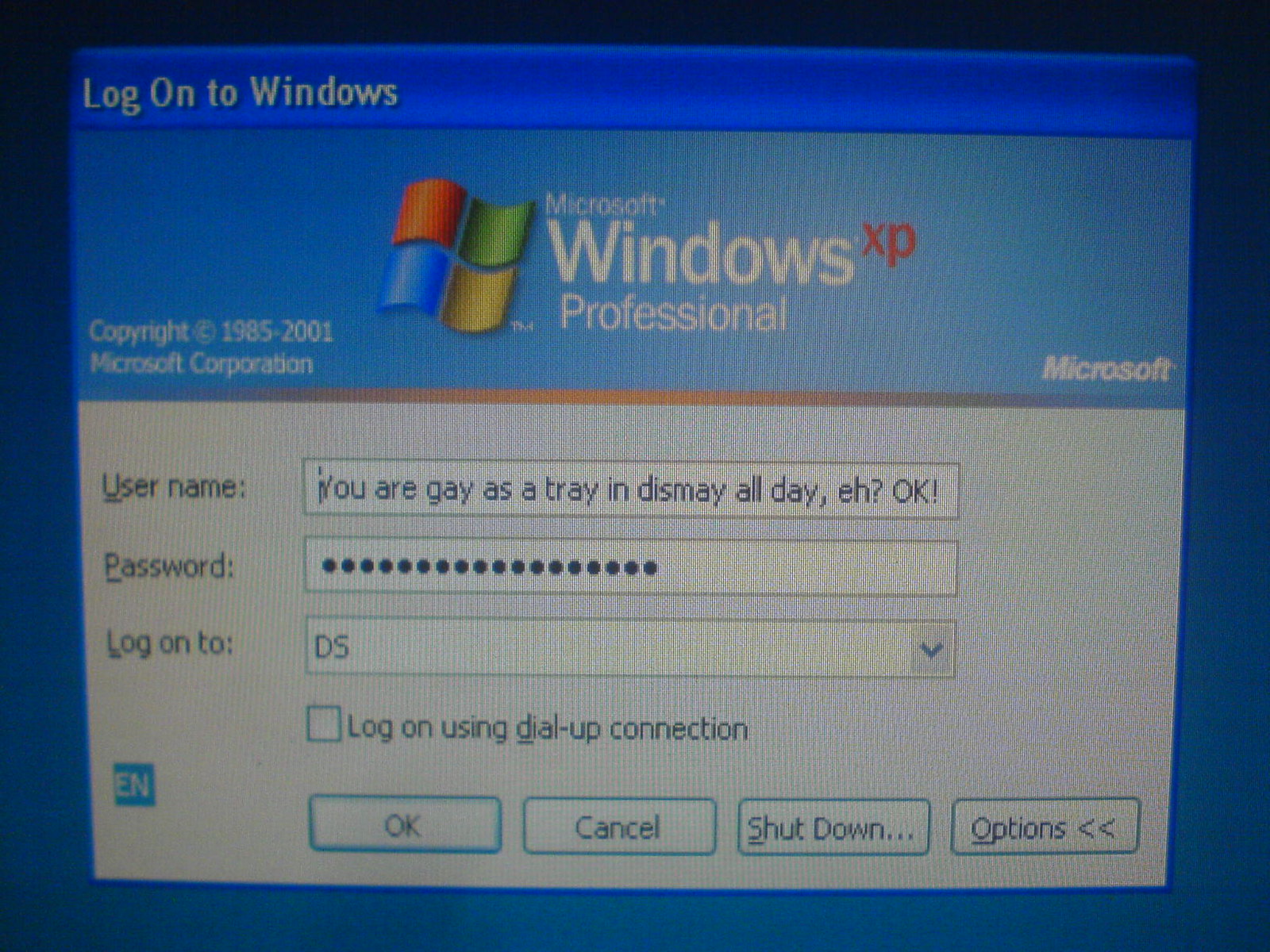This detailed photograph captures a computer screen showing the logon interface of Microsoft Windows XP Professional. Clearly taken with a camera, the image reveals scan lines across the screen. Centered at the top, the screen displays “Log on to Windows” along with the Microsoft Windows XP Professional logo, featuring its iconic red, green, blue, and yellow flag. Below this, the familiar logon interface includes a text box for the username, where the phrase "you are gay as a tray in dismay all day, A. Okay" is entered. The password field is filled with obscured dots for privacy. Adjacent to these fields, the screen shows “log on to DS” with a dropdown option. At the bottom of the screen, four buttons are aligned: OK, Cancel, Shutdown, and Options. Blue borders frame the login pane, encapsulating the vintage aesthetic of this Windows XP era.